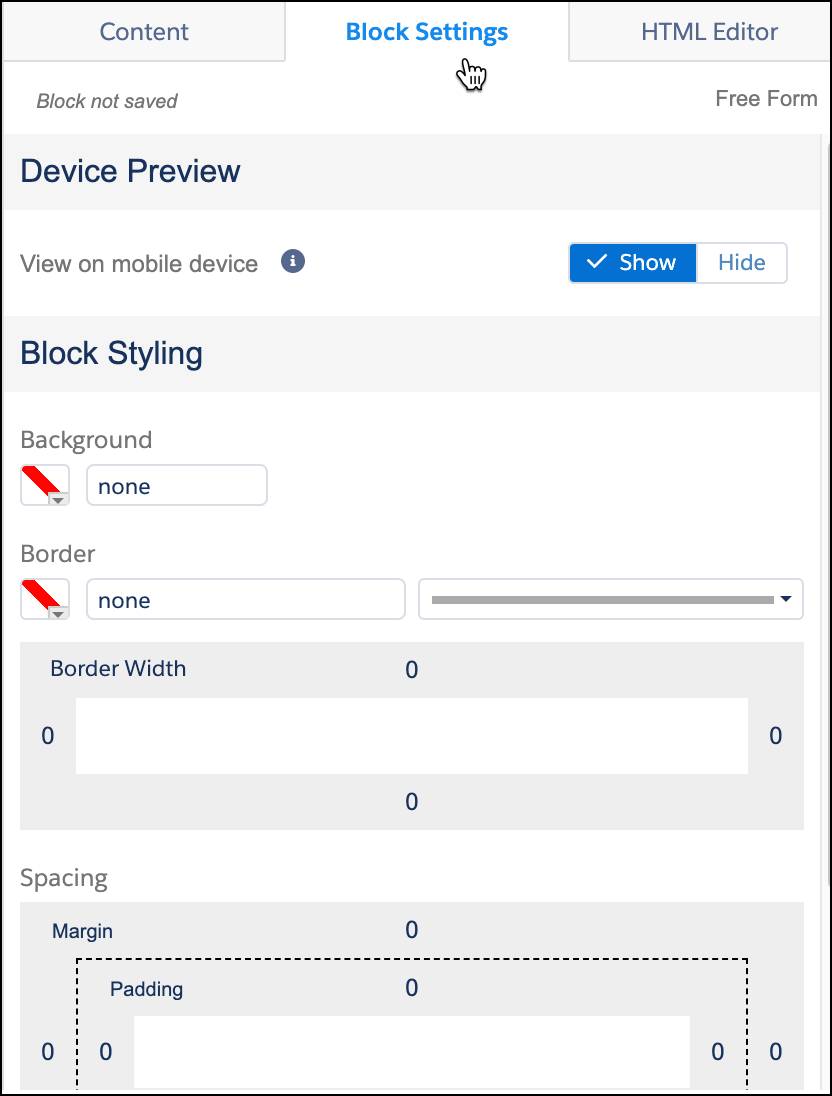The image depicts a user interface with a blue and white striped background. At the top, the word "Content" is prominently displayed. Below it, there are sections labeled "Block Settings" and "Blueprint," the latter indicated by a hand icon pointing upwards with its index finger extended. There is also an "HTML Editor" section, followed by a notification stating "Block Not Saved." To the right, there's a "Freeform" section.

Just below, there is a "Device Preview" feature, with options to "View on Mobile Device." This section includes a blue circle with an eye icon. Adjacent to this are the "Show" and "Hide" buttons, where the "Show" button is blue and the "Hide" button is white. 

Further down, the "Block Styling" section is visible, including a small block icon accented by a red dot. This section provides options to customize the "Background" (currently set to "None") and "Border" settings, also marked by a small red pin. An adjacent element, a box with a thick horizontal line and a down arrow, likely offers additional customization options.

Lastly, settings for "Border Width" and "Spacing" are shown, with all border widths set to zero. Both "Margin" and "Padding" parameters are similarly configured, each set at zero across the entire interface.